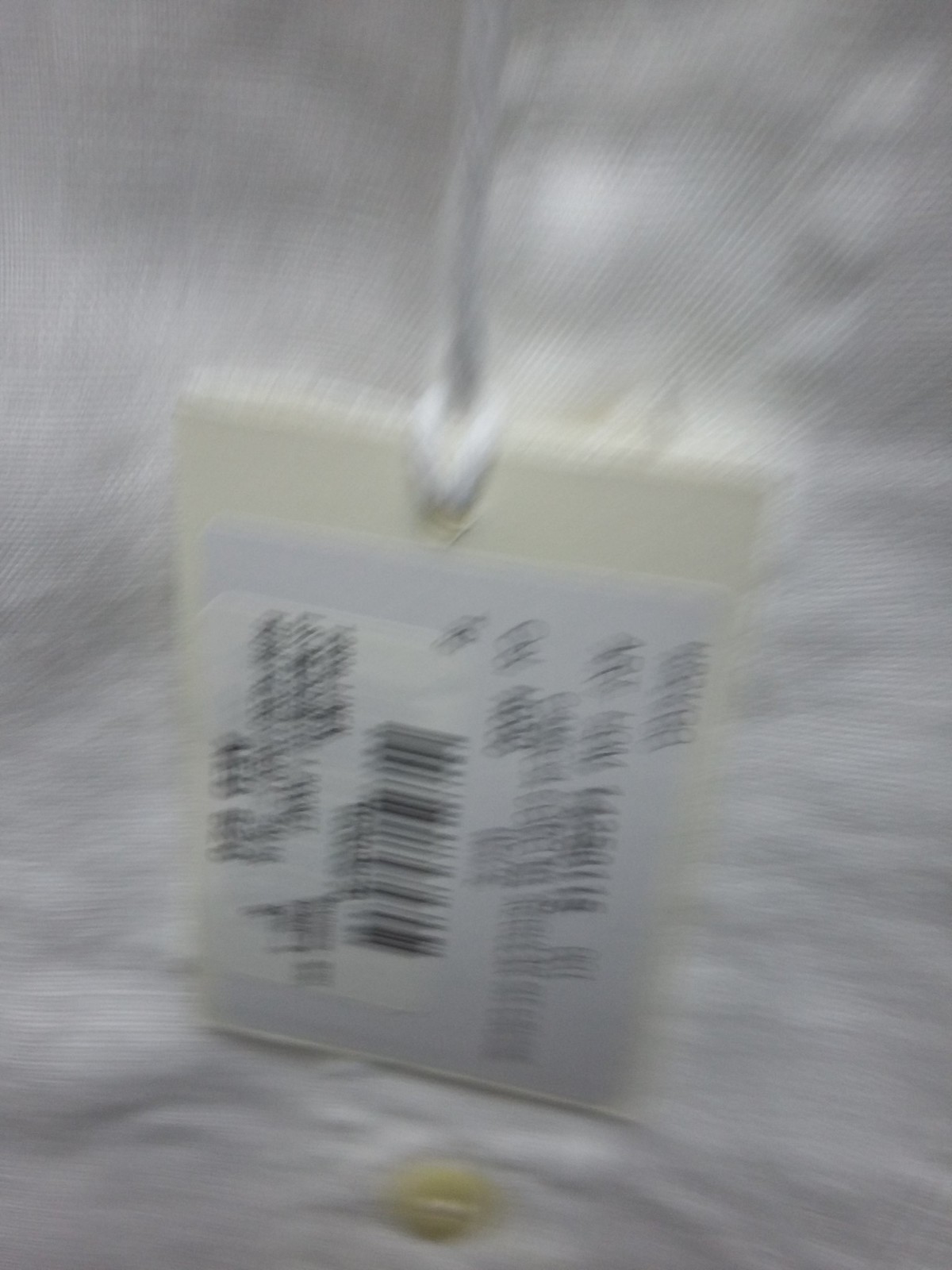The image is a highly blurry close-up of a beige tag, similar to those attached to items for sale. The tag is hanging by a string that loops through a hole at its top. Affixed to the tag is a white sticker, and there appears to be another white sticker partially overlapping it. The stickers display a barcode and a sequence of numbers, both of which are oriented sideways, indicating that the tag is dangling.

Despite the blurriness, some text is faintly discernible. The word "linen" and sequences of numbers including "4415," "0115," and possibly an address are visible, though indistinct. Additional text suggests the words "art," "hart," and "home." The background of the image has a shaded, pencil-like gray texture. At the bottom center, there is a yellowish smudge, adding a faint hint of color to the otherwise monochrome scene.